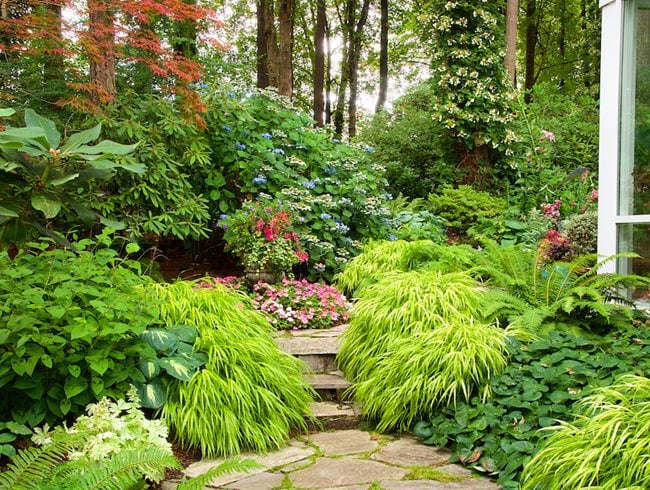The photograph captures a breathtakingly lush garden, reminiscent of something you might find in Better Homes and Gardens magazine. In the foreground, a half-circle stone walkway and a few stone steps lead through verdantly dense foliage. Nestled among the vibrant greens are flowering displays, including a wooden structure brimming with flowers. On the right side, a white pole-like structure with glass accents can be seen, possibly a bay window or porch pillar, hinting at the garden's domestic setting. The garden is alive with a variety of plants: dark and light green leaves, ferns, and bushy, grass-like vegetation. Colorful blooms of purple, red, white, pink, and blue burst through the green canvas. Tree trunks rise in the background, some adorned with white and reddish-orange leaves that add a splash of autumnal color to this sanctuary of natural beauty.